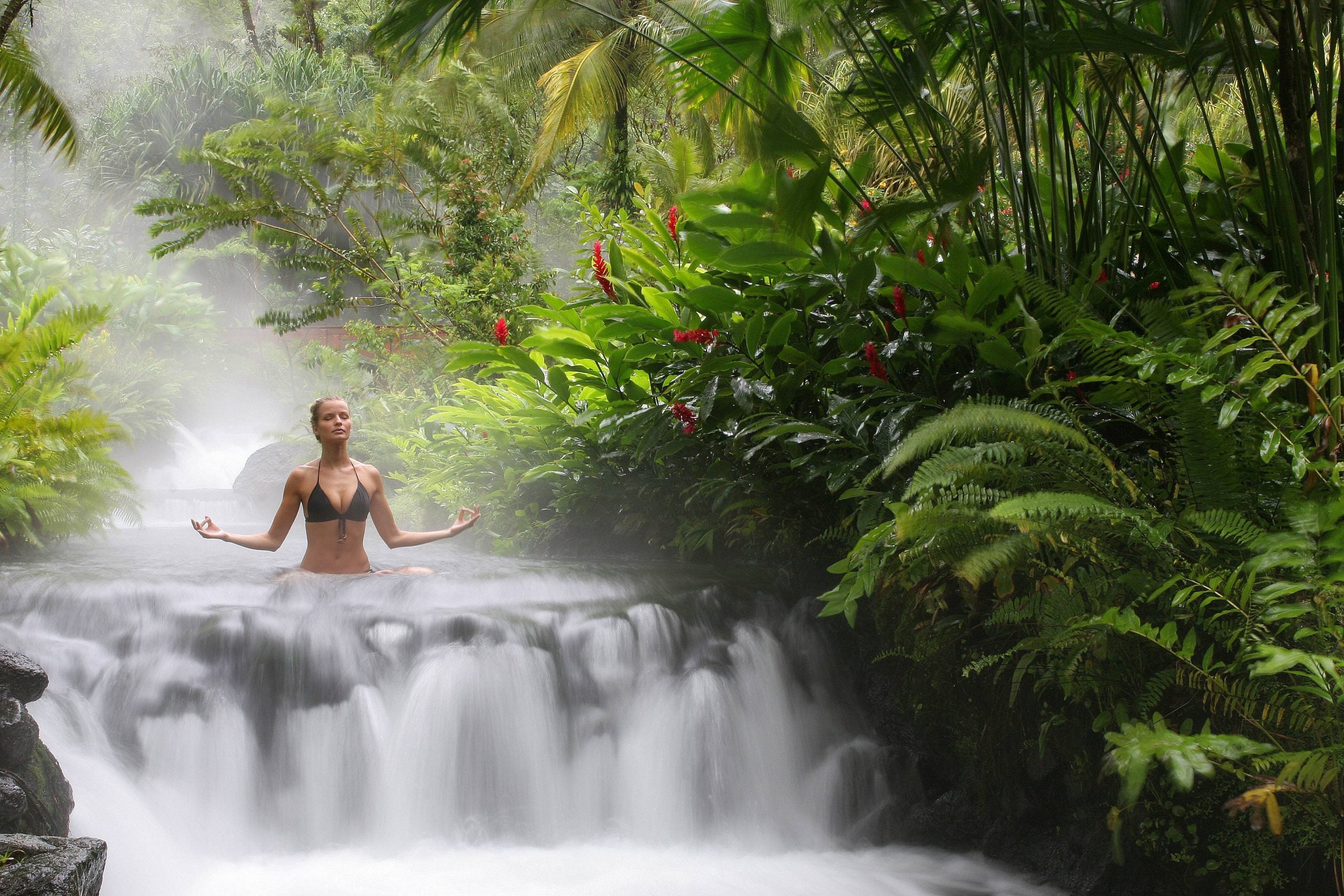The image depicts a serene scene set in a lush rainforest, centered on a small, shallow waterfall cascading down approximately three feet. Dominating this tranquil setting, a blonde woman sits cross-legged at the waterfall’s edge, meditating with her eyes closed and her face slightly tilted upwards. She has her hair pulled back into a bun and is dressed in a black bikini bathing suit, with her midriff exposed. Her arms are positioned outwards to her sides, hands lifted in a classic meditation pose with fingers forming a gentle V shape. She is surrounded by verdant, dense foliage, punctuated by vibrant pink and red tropical flowers. The bottom left corner of the image reveals a few rocks partially submerged in the water, adding to the natural ambiance. The overall composition, with the woman slightly to the left of the center, evokes a sense of mindfulness and tranquility, reminiscent of a scene one might find in a meditation or yoga-themed magazine.